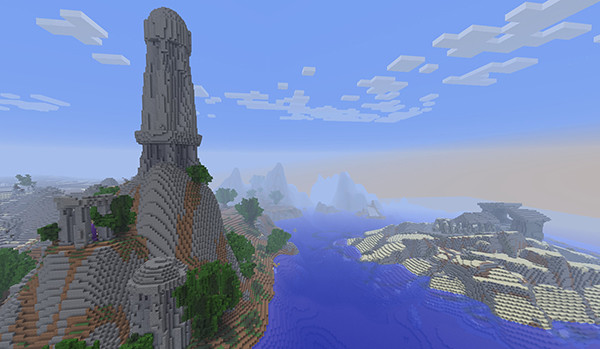A screenshot from the video game Minecraft captures a serene beach scene under a clear blue sky dotted with blocky white clouds. The distance is softened by a hazy ambiance, limiting the visibility into the horizon. In the foreground, a sandy beach extends into a body of deep blue water, out of which grow ancient-looking stone ruins. To the left, a grand gray-colored tower rises majestically into the sky, standing out against a brown and gray mountain backdrop. Below this tower, a smaller, ruin-like structure adds an element of mystery to the landscape.